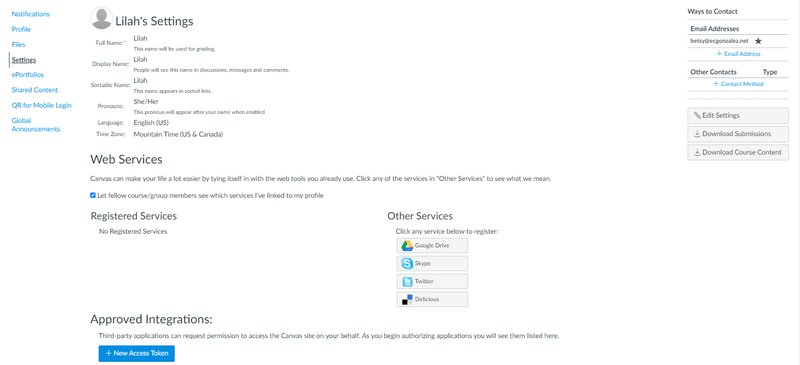**Caption: Detailed Screenshot of Lila's Account Settings in Canvas**

This screenshot captures the account settings page for a user named Lila in Canvas. On the left-hand side, there is a vertical menu with blue links, listed in the following order from top to bottom: Notifications, Profile, Files, and Settings. The "Settings" link is highlighted in black, underlined, and accompanied by a black vertical bar, indicating the current page. Below this are additional links for ePortfolios, Shared Content, QR for Mobile Login, and Global Announcements.

In the main section of the page, a placeholder gray circle represents Lila’s profile picture. The header reads "Lila’s Settings," followed by detailed information:

- **Full Name**: Lila (This name is used for grading purposes).
- **Display Name**: Lila (Visible to others in discussions, messages, and comments).
- **Sortable Name**: Lila (Used in sorted lists).
- **Pronouns**: she/her (These pronouns appear after the name when enabled).
- **Language**: English (U.S.).
- **Time Zone**: Mountain Time (U.S. and Canada).

A section titled "Web Services" explains how Canvas can integrate with other web tools to enhance user experience. There is a small blue square with a white check mark labeled "Let fellow course/group members see which services I've linked to my profile."

Under "Registered Services," it states "No registered services." The "Other Services" section invites Lila to register services such as Google Drive, Skype, Twitter, and Delicious.

Following "Web Services," the heading "Approved Integrations" describes how third-party applications can request access to Lila's Canvas account, listing them once authorized. A blue rectangle labeled "New Access Token" is available for generating tokens.

On the right-hand side, the "Ways to Contact" section is outlined with a gray line, listing an email address: Betsy at ccgonzalez.net, accompanied by a black star. Additional contact methods can be added via blue plus signs for email and other contact methods. Finally, three gray rectangles provide options for "Edit Settings," "Download Submissions," and "Download Course Content."